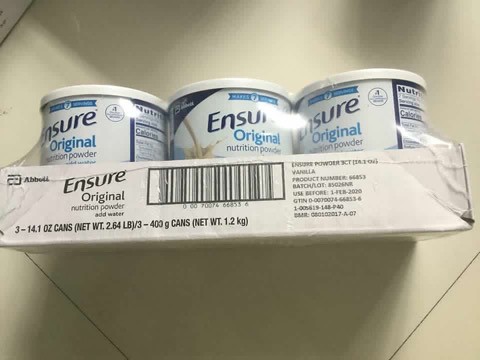This is a detailed photograph of a sealed package of Ensure original nutrition powder, taken on a white or cream-colored tiled or linoleum surface. The package consists of a small white cardboard tray holding three 14.1-ounce cans (403 grams each, total net weight 1.2 kilograms). Each can is white with dark blue "Ensure" branding and lighter blue text detailing "original nutrition powder." The cans are arranged in the tray and wrapped in clear plastic shrink wrap, although they are not perfectly aligned. The wrap is tight and covers the entire product, ensuring it remains sealed. Additional information is printed on the packaging, such as nutrition details, batch code, product number, and an ISBN-like barcode. The tray, designed for retail display, indicates it's a shop-ready package that could either be unpacked and stocked on shelves or sold as a complete unit. The writing also mentions vanilla flavor and includes an expiration date of "before 1 February 2020," along with the manufacturer's name, Abbott.